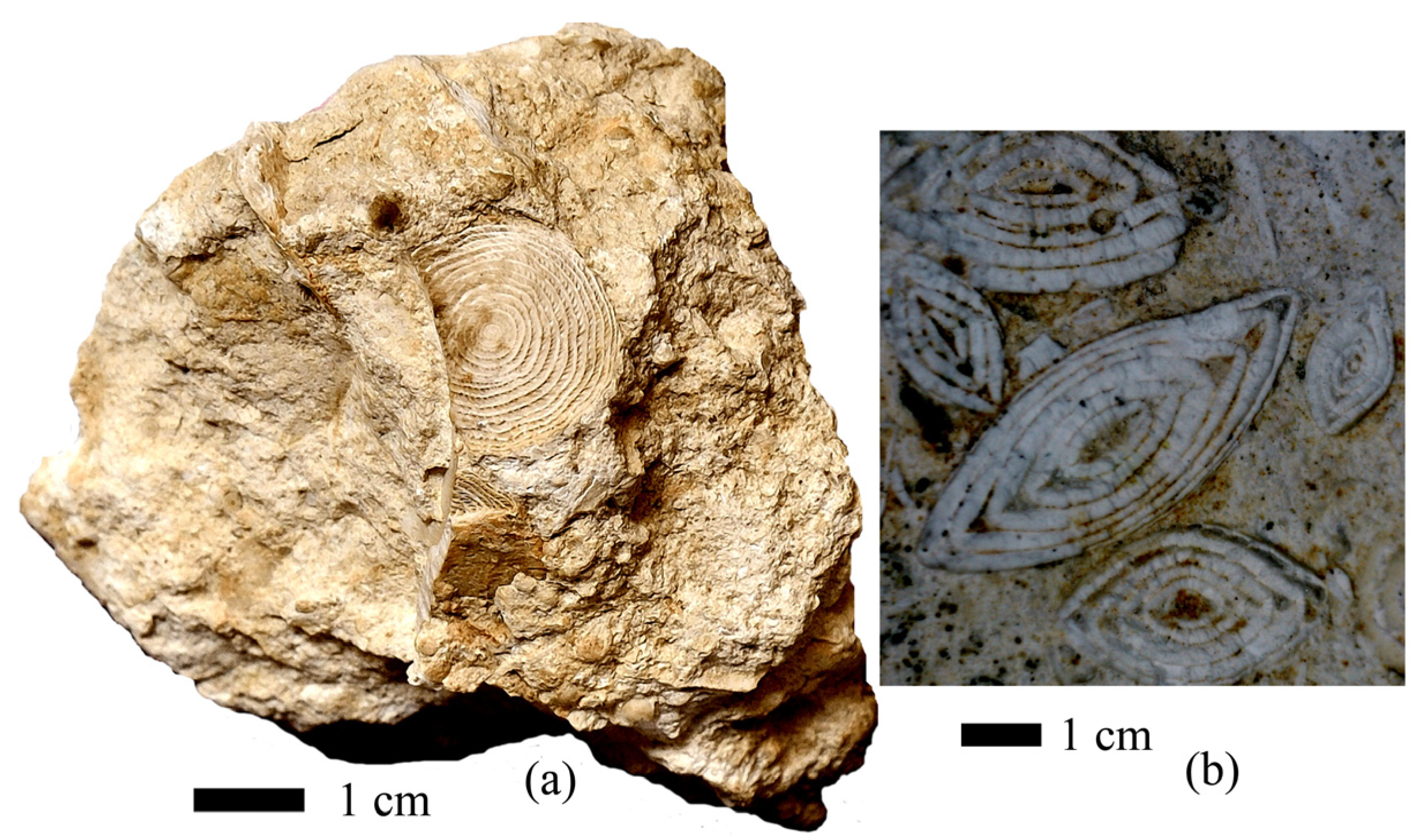The image captures a detailed view of a rock and its fossilized texture, divided into two distinct figures labeled "A" and "B". Figure A, on the left, showcases the overall appearance of the rock, which is predominantly an orange-brown or tan hue with a rough, ridged exterior. At its center, there is a prominent circular pattern consisting of about 10 to 12 concentric rings. The rock itself has an irregular, multifaceted shape and is accompanied by a scale bar beneath it indicating "1 cm" in black text, with the letter "A" in parentheses next to it.

Figure B, on the right, presents a microscopic close-up of the rock's texture, highlighting oval or eye-shaped patterns within the fossilized structure. These shapes are layers of smaller ovals nested within each other, resembling cross-sections of an onion, and are colored in shades of white, tan, and black with speckled details. Similar to Figure A, a black rectangle beneath the image denotes a "1 cm" scale bar, followed by the letter "B" in parentheses. The background of the image is white, providing a clear contrast to the fossil's intricate patterns.